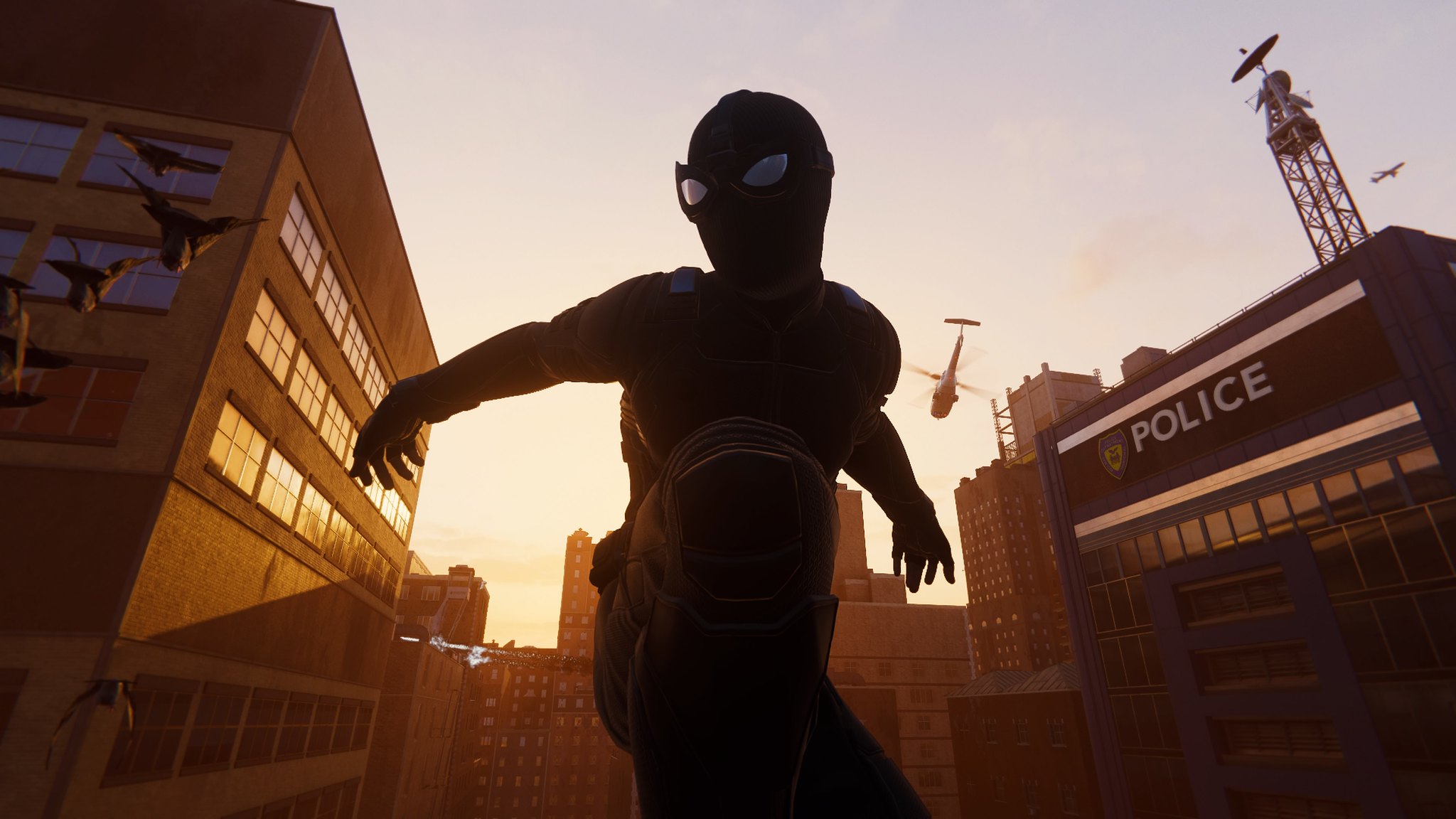In this detailed photograph of a screenshot from a Spider-Man video game, a central character, resembling Spider-Man with distinct white, bug-like eyes, is prominently featured. His pose and attire give the impression of a superhero, seemingly flying, with much of his detailed costume obscured in shadow, implying he might be wearing black. To the right of the character, a large building displays the word "POLICE" in white with a police badge emblem, suggesting a police department similar to New York City's. Behind this building, a helicopter is flying away. On the left side, another building is illuminated by the setting sun, enhancing the scene with a warm, sunset glow. Birds are seen flying across this building, adding to the dynamic background. Additionally, an antenna with a satellite dish is visible in the upper right corner, and far in the distance, a commercial passenger plane is in flight, completing the intricate urban panorama.